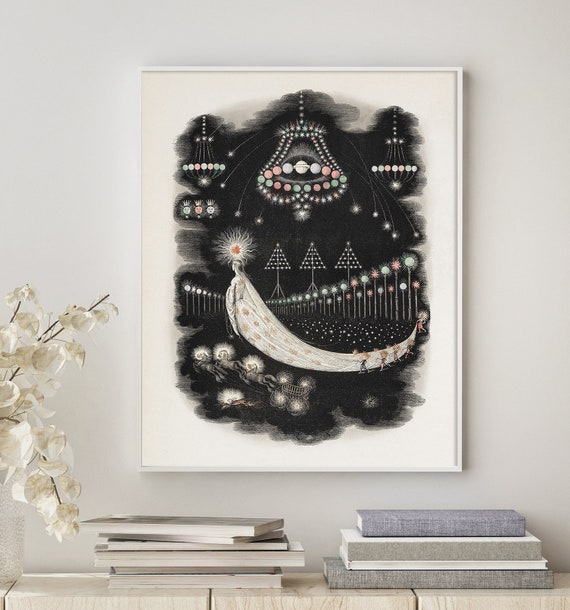The photo displays a painting hanging on a cream-colored wall, which is framed and matted in white. The painting itself has a black background and showcases an abstract depiction of a woman wearing a long, white gown, held up by several people. Above her head, there are multiple chandeliers with lights that appear white, pink, and light green, resembling glowing orbs or planets. The painting includes other abstract elements like three triangular shapes that could represent stylized Christmas trees made out of circles. Below the painting, there is a table or buffet adorned with stacks of books. On the left side, there are five or six books displayed with their pages facing outward, while on the right side, there are four books with their spines toward the viewer. Additionally, there's a white plant next to the books, contributing to the overall white aesthetic of the setup.